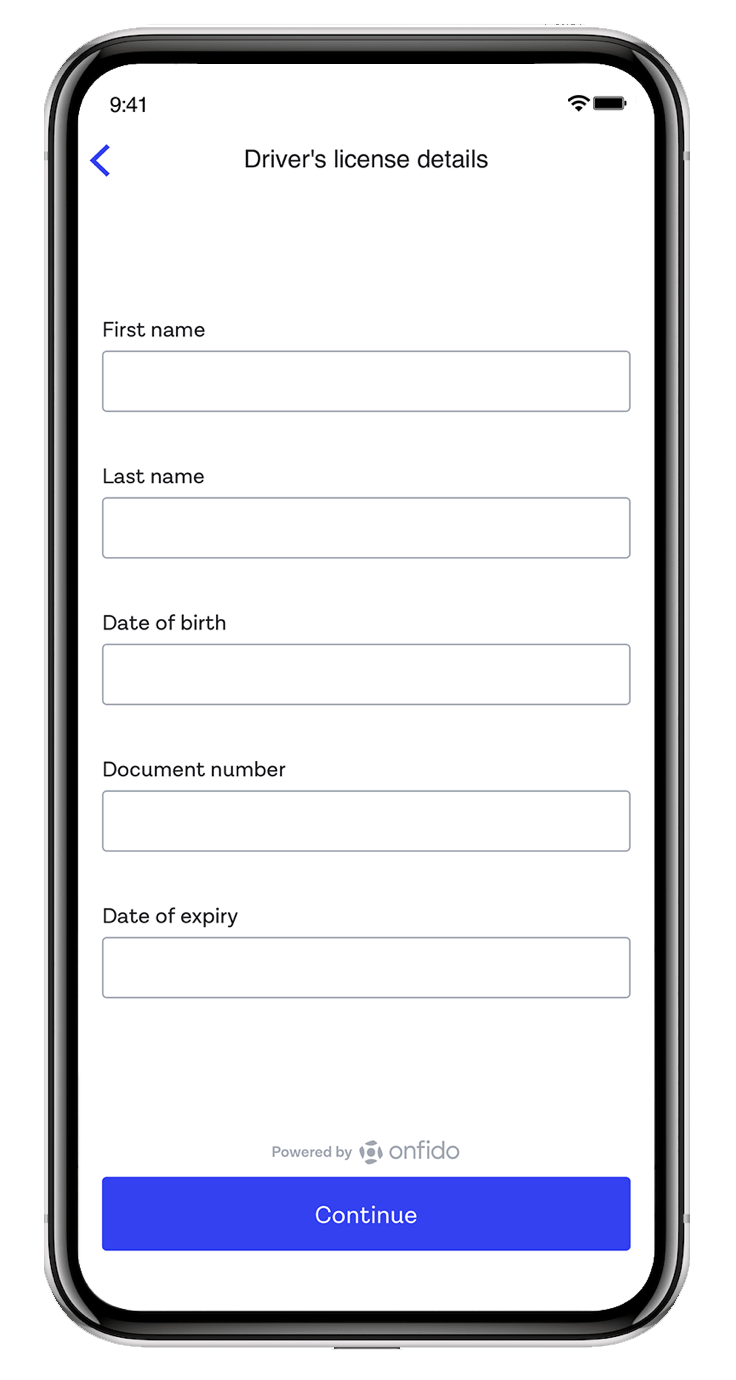**Detailed Caption:**

The image depicts the front screen of a smartphone showing an app interface, likely dedicated to updating or saving driver's license information. The top section displays the time as 9:41, with a full Wi-Fi signal and battery icon indicating the device is well connected and charged. Just below the time, a blue arrow icon pointing left is visible, symbolizing a 'Back' function. Centered at the top of the screen, the heading "Driver's License Details" is prominently displayed.

The main interface comprises multiple text input fields, each outlined in grey with a white background inside. The first field is labeled "First Name," followed by a corresponding text box. Directly below is another field labeled "Last Name," accompanied by another text box. The subsequent fields include "Date of Birth," "Document Number," and "Date of Expiry," each paired with their respective boxes for input. All labels are written in black, ensuring readability.

At the bottom right corner of the screen, "Powered by Onfido" is indicated, suggesting the verification service used by the app. The bottom part of the interface features a distinct blue button with the word "Continue" inscribed in white, guiding users to proceed with their input.